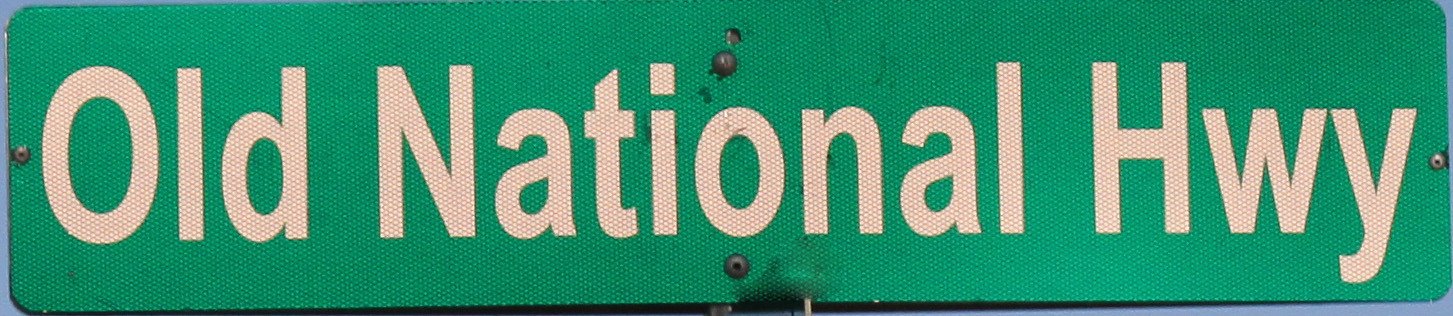This is a very close-up photograph of a weather-worn street sign with a green background and reflective white letters. The sign reads "Old National HWY" with the first letters capitalized. The center of the sign features a large, dark gray, and black rivet or weld above the "O" in "Old," accompanied by a smaller rivet nearby. Below the "O," there is noticeable damage, including a large weld mark and a dent, causing the paint to bubble. The sign is affixed with silver screws or rivets at the left and right center edges. The edges of the sign reveal an overcast, dark blue sky. The sign appears rectangular and slightly bent below the "O" in "Old", giving it a well-used and aged appearance.